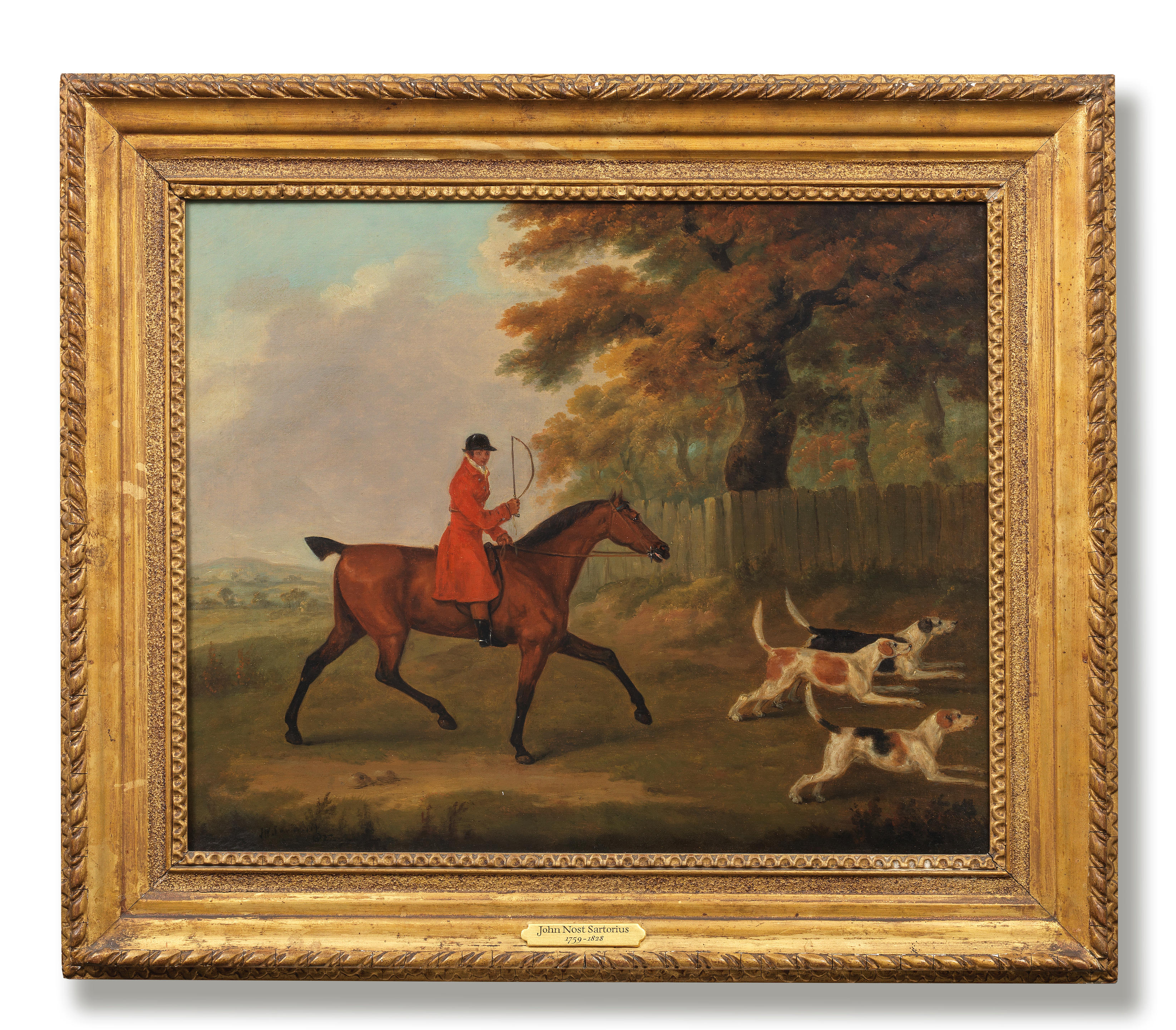This rectangular image, about four inches high and five inches wide, captures a photograph of an old, traditionally framed painting, set against a white wall. The painting is encased in a thick, chunky, gold-colored frame featuring ornate gold leaf vines, which casts a noticeable shadow on the wall. The frame includes a small plaque at the bottom center, bearing the name John Knost Sartorius, along with his dates, 1759 to 1828.

The artwork itself depicts a quintessential English countryside scene: a fox hunter dressed in a vivid red coat and traditional black horse riding cap. The hunter is mounted on a well-manicured brown horse with a black mane and a neatly cropped tail, holding a whip in their right hand. Three slender hounds, predominantly white with black and brown patches, race ahead of the horse. In the background, there's a low wooden fence and large trees, with an expansive open valley stretching to the left under a sky painted with shades of blue and gray clouds. The detailed illustration evokes a vivid sense of a classic fox hunting expedition.